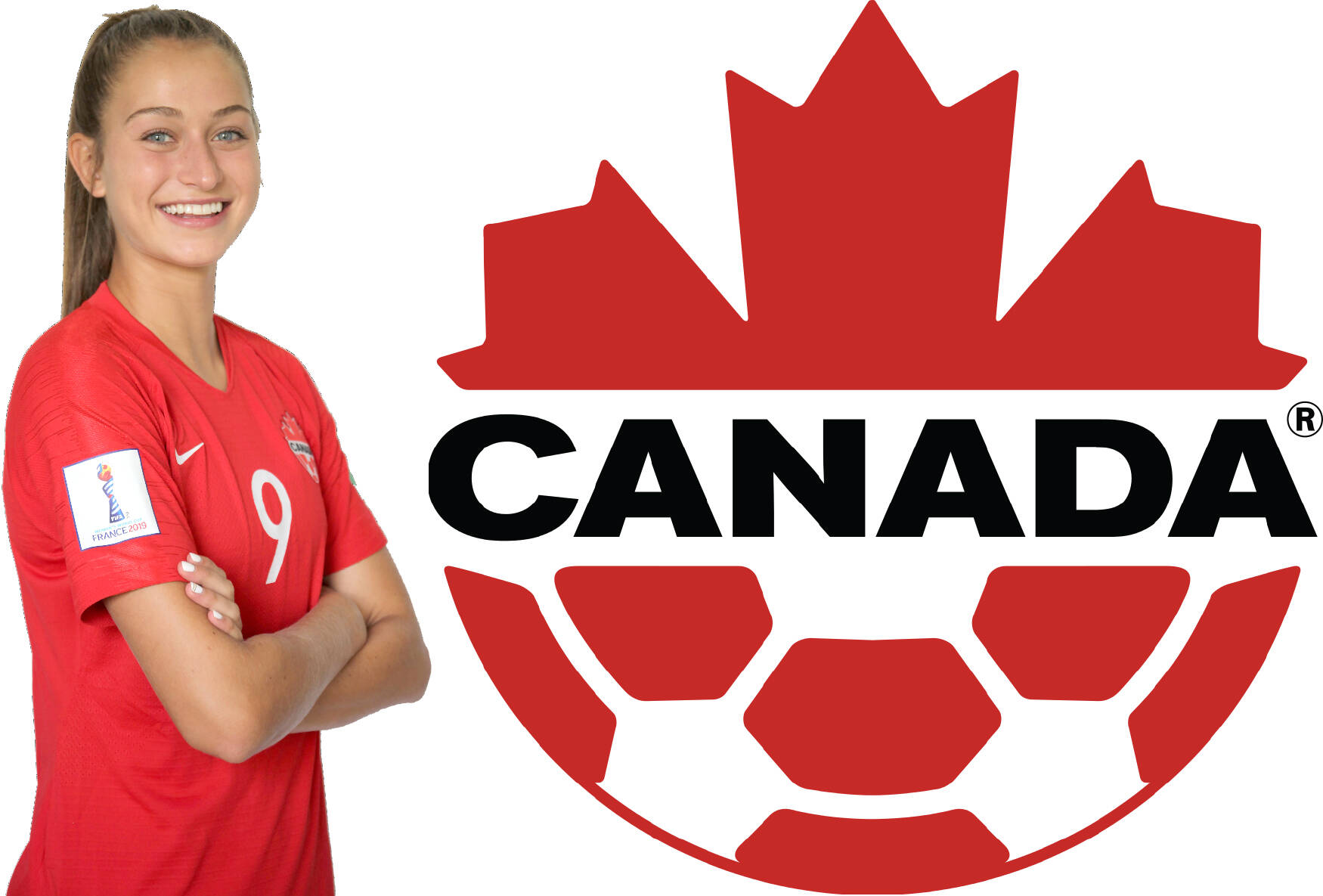This image captures a young woman, likely a soccer player, positioned on the left side. She has long brown hair pulled back into a ponytail, blue eyes, and she is smiling directly at the camera. She is dressed in a red Nike shirt with her arms crossed, and the shirt prominently features a white number nine at its center. On her right shoulder (the left side of the image), there's a white square patch that reads "France 2019," adorned with an Olympic-style flame. Additionally, another unspecified logo is visible on her shirt. A distinct logo is printed to the right of her in the image, featuring the word "Canada" in bold black letters. The logo is divided into two parts, with a red soccer ball's bottom half and the Canadian maple leaf's top half, suggesting it is likely the Canadian World Cup logo.